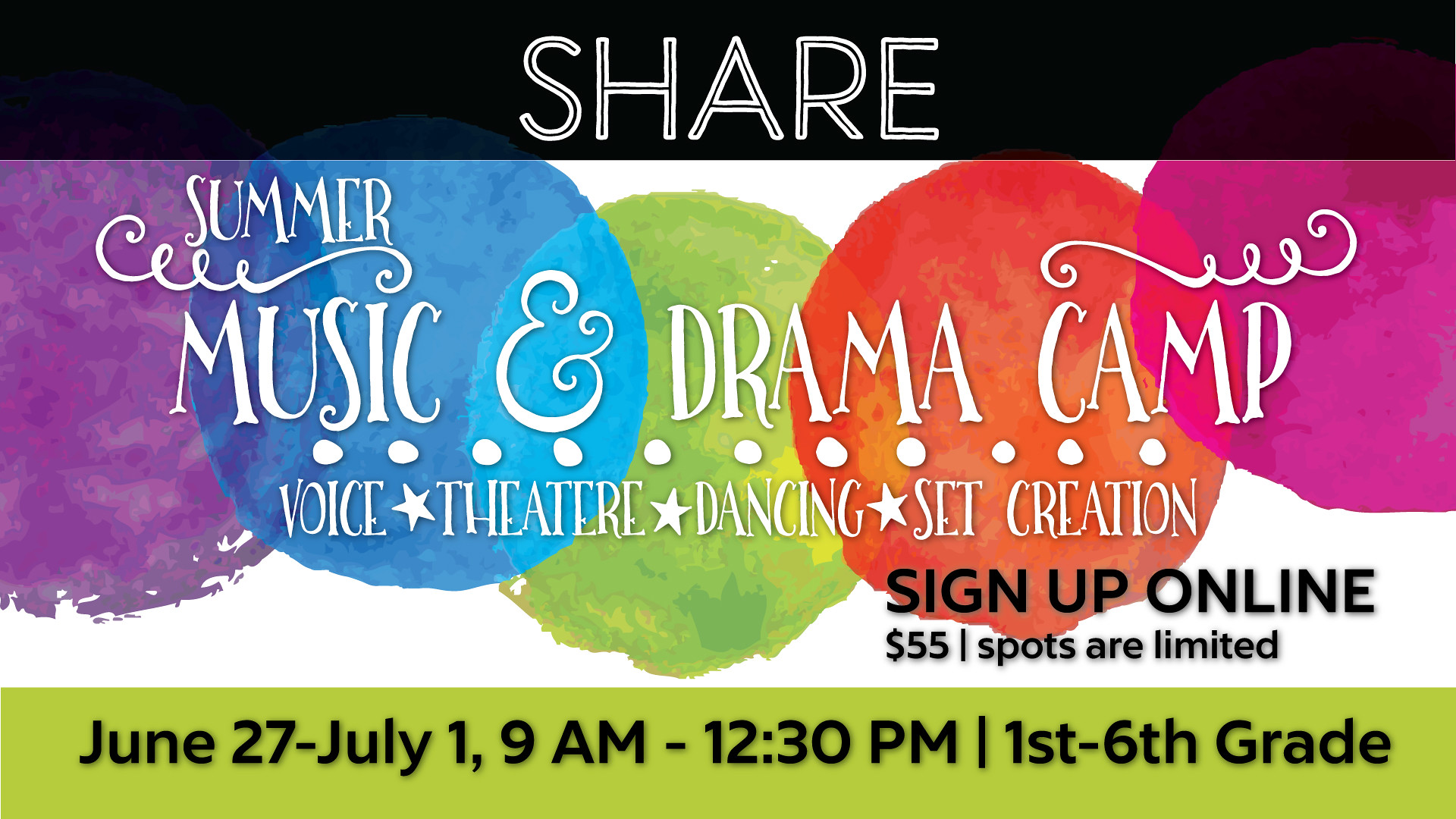The image features a banner promoting a summer music and drama camp. At the top, a slightly transparent black bar spans the width of the design, with the word "SHARE" displayed prominently in large white letters. The central portion of the graphic has a clean, white background adorned with overlapping circular blobs in a spectrum of colors—purple, blue, green, orange, and a second shade of purple—resembling paint splatters. Superimposed over these vibrant blobs are the words "SUMMER MUSIC AND DRAMA CAMP" followed by "VOICE, THEATER, DANCING, SET CREATION" in crisp white letters. Towards the bottom right of this area, there's a note that says "Sign up online for $55. Spots are limited," in black text. The base of the image features a slim lime green strip with black text that provides the camp details: "June 27th - July 1st, 9 a.m. - 12:30 p.m., first through sixth grade." This promotional piece resembles a digital card or an online invitation, exuding a fun and energetic atmosphere for a creative summer experience.